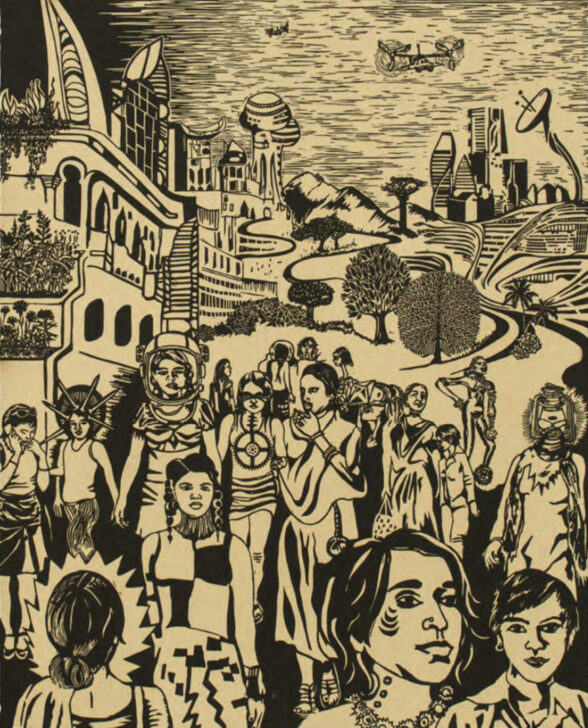This detailed illustration, rendered in black and sepia tones, captures a complex scene featuring a diverse group of people gathered in the foreground against a backdrop of various buildings and landscapes. The background is filled with a mixture of futuristic structures, classical buildings, trees, and what appears to be water and a ship at the edge of the horizon. There's also a satellite dish and something flying in the air, adding a layer of modernity and intrigue.

In the foreground, the people are depicted with intricate detail, each sporting unique outfits and distinct features. Noteworthy characters include a person with spikes resembling the Statue of Liberty's headdress, wearing a tank top, and another person donning a space helmet paired with a dress. Some figures are more subdued, such as a person in a robe and another with a collared shirt staring straight ahead. A woman in a beekeepers' hat holds a little boy's hand at the leftmost corner, while another woman with hair tied back in a bun has her back turned to the viewer. A person with lines painted on their face and a necklace stands out among others, while another wears a sari and yet another a fur hat. The diversity in attire and appearances highlights the eclectic nature of this assembly, each individual adding to the rich tapestry of the scene.